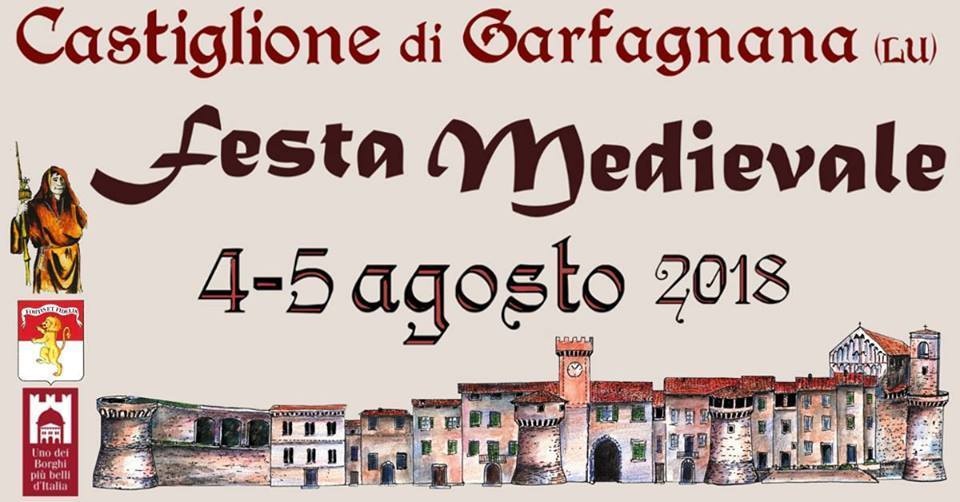This rectangular poster advertisement for the "Festa Medieval" has a rich and detailed design. The backdrop is a muted brownish-gray color, setting a historical tone. At the top, maroon text prominently announces "Festa Medieval," followed by the dates "4-5 Augusto, 2018" in the same maroon hue, with additional text, "Castiglione di Garfagnana" and "Lou" in brackets. The text appears to mimic a Latin style of writing.

The bottom section of the poster features an illustrated graphic of a medieval town with several interconnected buildings, arched doorways, and a dominant clock tower at the center. The structures evoke the architecture of old medieval times, complete with turrets and towers.

On the left side of the poster, there is a striking figure of a woman with an elfish face, red hair, and a brownish-red robe. She holds a gold staff, adding a mythical element to the scene. Below her figure is a notable red and white flag depicting a gold lion in the middle and a white banner above it, further enhancing the medieval theme.

At the bottom left corner, there is a maroon rectangular logo with white accents, adding a modern touch to the traditionally themed poster. Additionally, there's a segment of text that reads, "Una del Borghel, Plu, Bel, Cetalia," possibly highlighting a significant aspect of the festival or its historic context. This comprehensive design vividly captures the essence and allure of the "Festa Medieval," enticing viewers with its detailed and immersive representation.